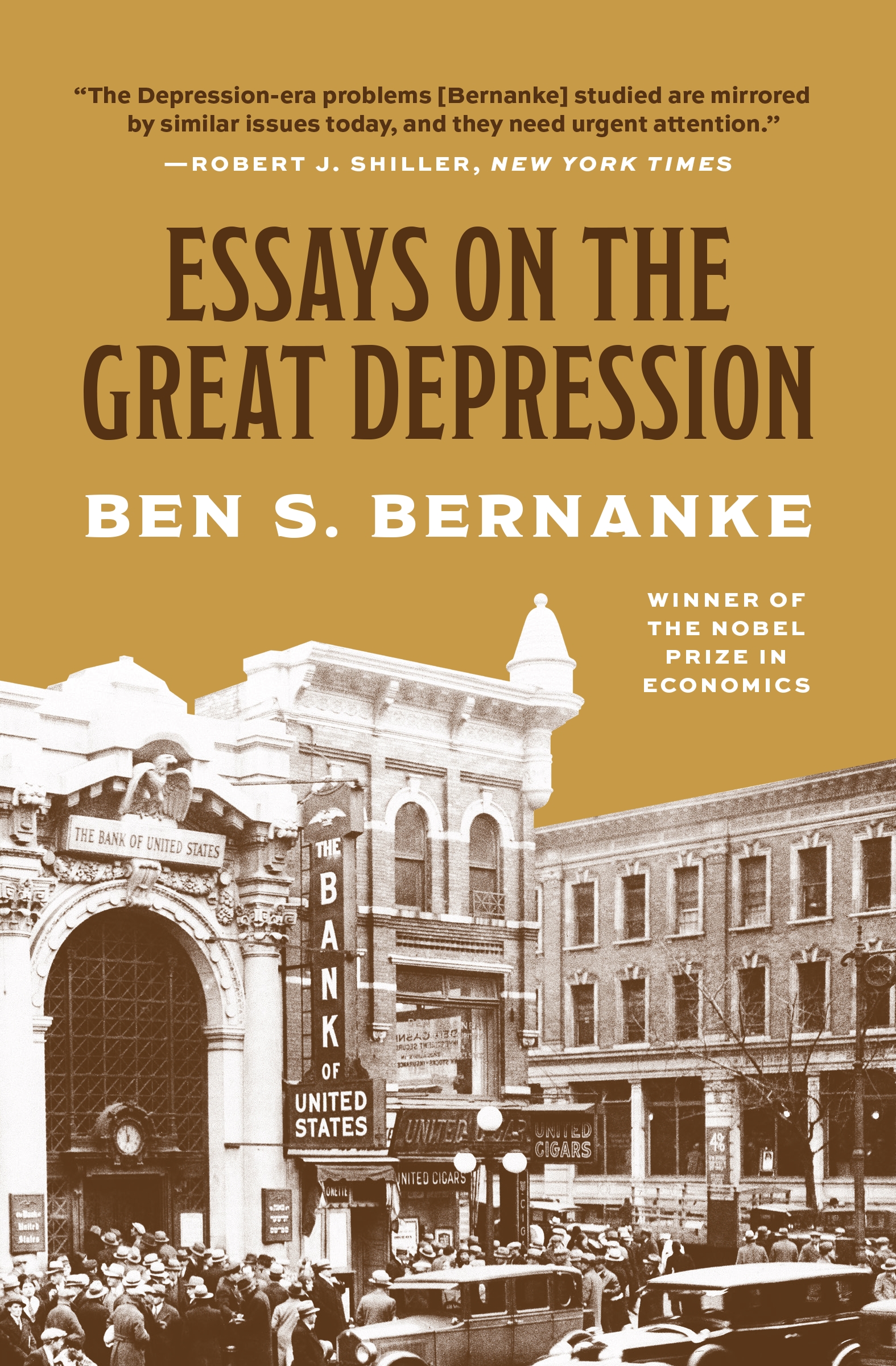The cover of the book "Essays on the Great Depression" by Ben S. Bernanke prominently features a sepia-toned, monochrome photograph from the Depression era. The image captures a bustling scene in front of the Bank of the United States, likely from the 1930s or 1940s, characterized by old-fashioned cars and a large crowd gathered outside. Above this historical cityscape, the title "Essays on the Great Depression" appears in bold black letters, with the author's name, Ben S. Bernanke, in white below it. Additionally, a small accolade in the lower right corner proudly notes that Bernanke is a "Winner of the Nobel Prize in Economics." The background is a simple, flat mustard color, accentuating the starkness of the photo and the text. At the top, a quote by Robert J. Schiller from the New York Times is displayed, emphasizing the relevance of Depression-era issues to contemporary economic challenges and their urgent need for attention.